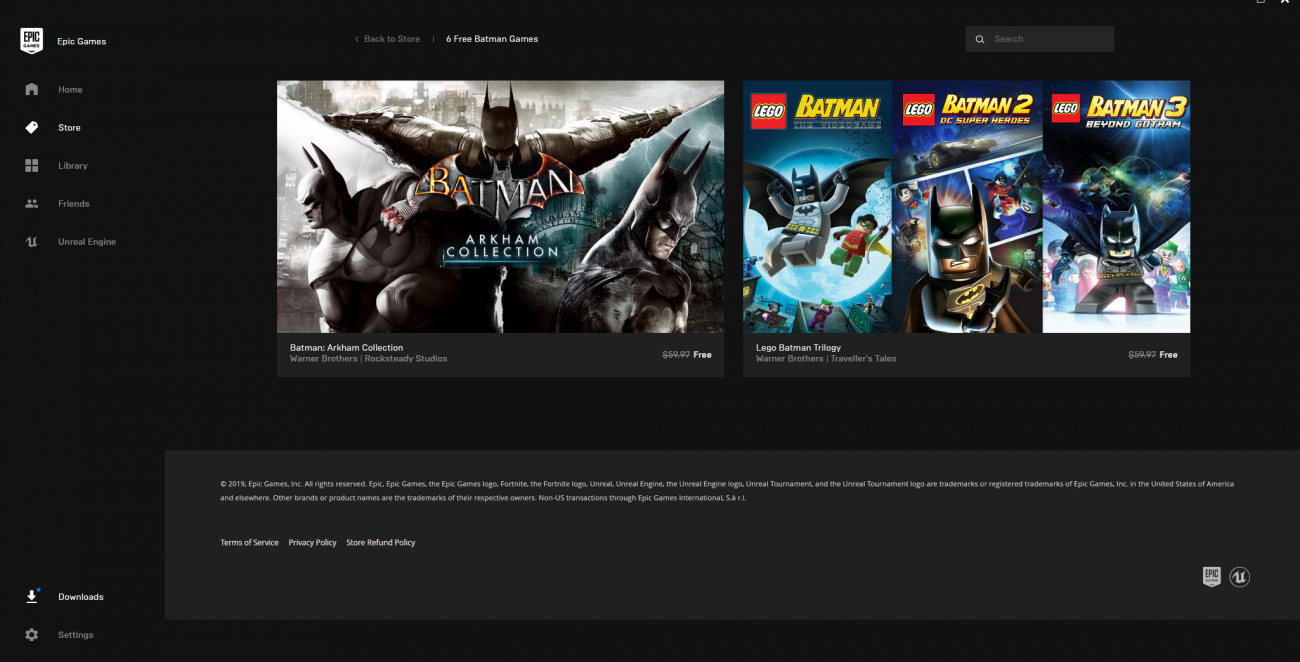The image depicts a screenshot of the Epic Games Store interface, framed by a black rectangular border, twice as wide as it is tall. In the top left corner is the Epic Games logo, featuring a black shield emblem with "Epic" in white text, and underneath in smaller lettering, "Games." To the immediate right, the text "Epic Games" is prominently displayed.

Below the logo, there is a vertical menu starting with a grey home icon accompanied by the text "Home." Next, a white store icon is labeled "Store," followed by a grey library icon labeled "Library," a friends icon labeled "Friends" in grey text, and a "U" icon with the text "Unread Engine" to the right. In the bottom left corner, a white download icon with a small blue dot next to it signifies active downloads, labeled "Downloads." Underneath, a grey settings icon is paired with the text "Settings."

Across the top, slightly left of center, there is a navigation link that reads "Back to the Store." Below this, a banner announces "6 for you Batman games."

On the right side, a grey search bar with a white search icon inside includes the word "Search." Beneath the "Back to Store" link, there is a large rectangular section featuring the "Batman Arkham Collection." This section prominently displays Batman imagery on both the left and right sides, and includes the title, the name of the developer, and the price on the right. Below are small thumbnails for "Arkham 1," "Batman Legos," "Batman 2," and "Batman 3 for Legos," with additional details and prices beneath.

Approximately three-quarters of the way down the page, there is a lighter black border enclosing two lines of detailed information about the games. At the very bottom, the footer contains links for "Terms of Service," "Privacy Policy," and "Store Reformed Party Policy" in white text. On the right side of the footer, the Epic Games logo is visible beside a black circle featuring a silver "U" with a silver border.